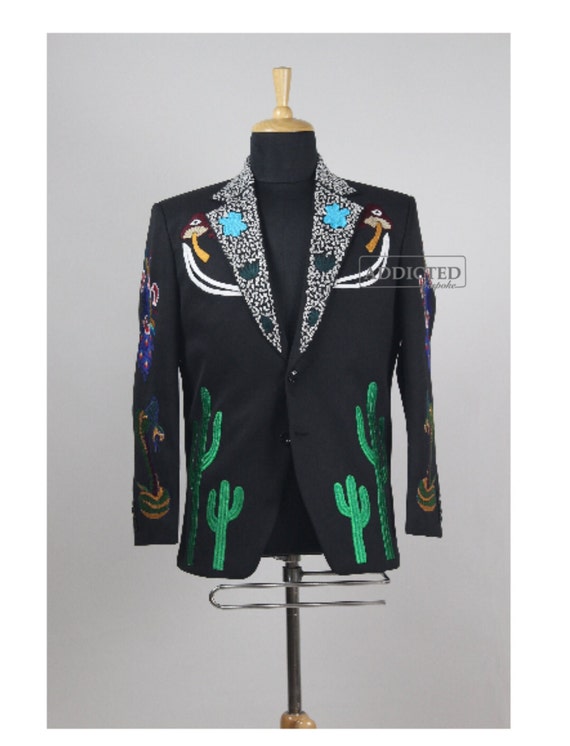The image is a detailed photograph of a black men's blazer, displayed on a headless mannequin against a medium gray background. This visually striking blazer features intricate, colorful embroidery and embellishments, making it a standout piece. On both the left and right sides of the jacket are large, embroidered saguaro cacti, while each sleeve showcases elaborate designs, including peacock motifs intertwined with snakes. The collar is adorned with white embroidery featuring blue flowers and green leaves. The chest area is decorated with two embroidered mushrooms, each topped with a small, red cap that gives a whimsical touch. The jacket also features black and white speckles on the wide lapels, adding to its unique charm. In the backdrop, a small gray box with the word "addicted" is faintly visible, situating the blazer in an artistic and fashionable context.